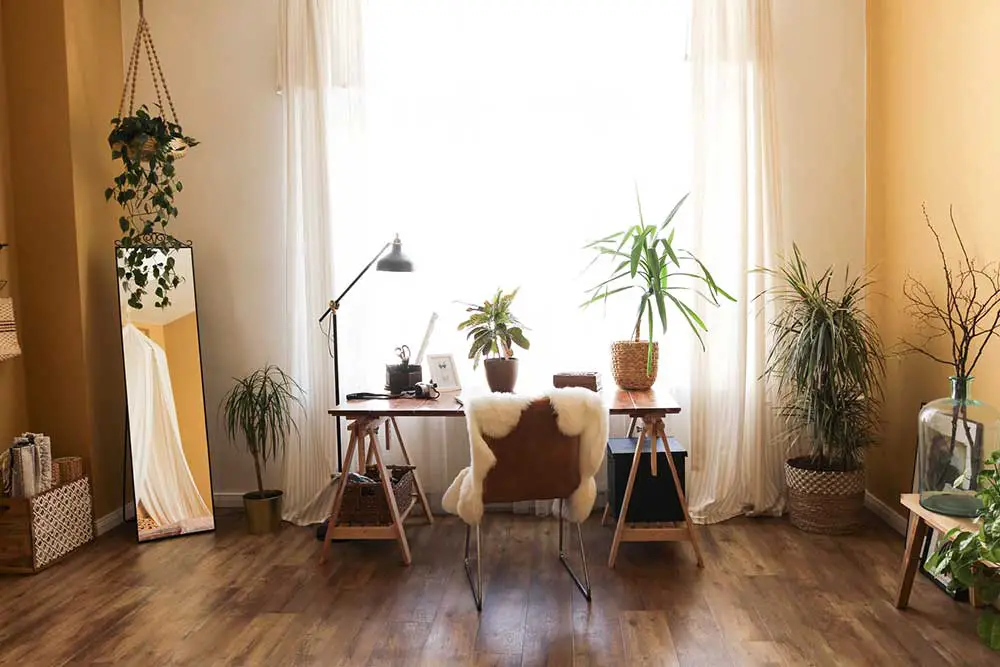The image captures a bright, modern room with a pristine hardwood floor and beige walls, showcasing a tidy workspace centered in front of a large, sunlit window draped with thin white curtains. The wooden desk, supported by triangular sawhorse-like legs, features two plants - a small one and a taller plant in a light wicker basket. On the left side of the desk, you can spot a lamp, a camera, scissors, and a photograph in a picture frame. A brown chair with metal legs and a white, furry covering sits in front of the desk. To the left of the desk is a large, rectangular floor mirror with a hanging plant above it. Additional plants in pots decorate both the left and right sides of the room. The scene is bathed in natural light, creating a bright and inviting atmosphere.